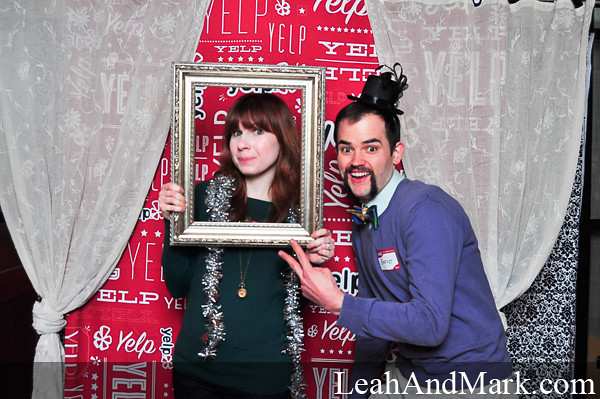The image depicts an indoor setting at what appears to be a Yelp event, based on the red step-and-repeat backdrop adorned with the Yelp logo. The backdrop is flanked by tied white curtains on both sides. In the center-left of the image stands a woman with dark hair and pale skin, dressed in a black outfit complemented by a green sweater. She is adorned with a silvery tinsel scarf and a gold pendant necklace. The woman is holding up a picture frame around her face. To her right is a man with a distinctive mustache and beard, wearing a purple sweater over a collared shirt, paired with a bow tie. He sports a small, black miniature hat on his head. The man is making a peace sign with his left hand towards the woman while also helping to hold the picture frame. The lower right corner of the image features the text "leahandmark.com" in white lettering.